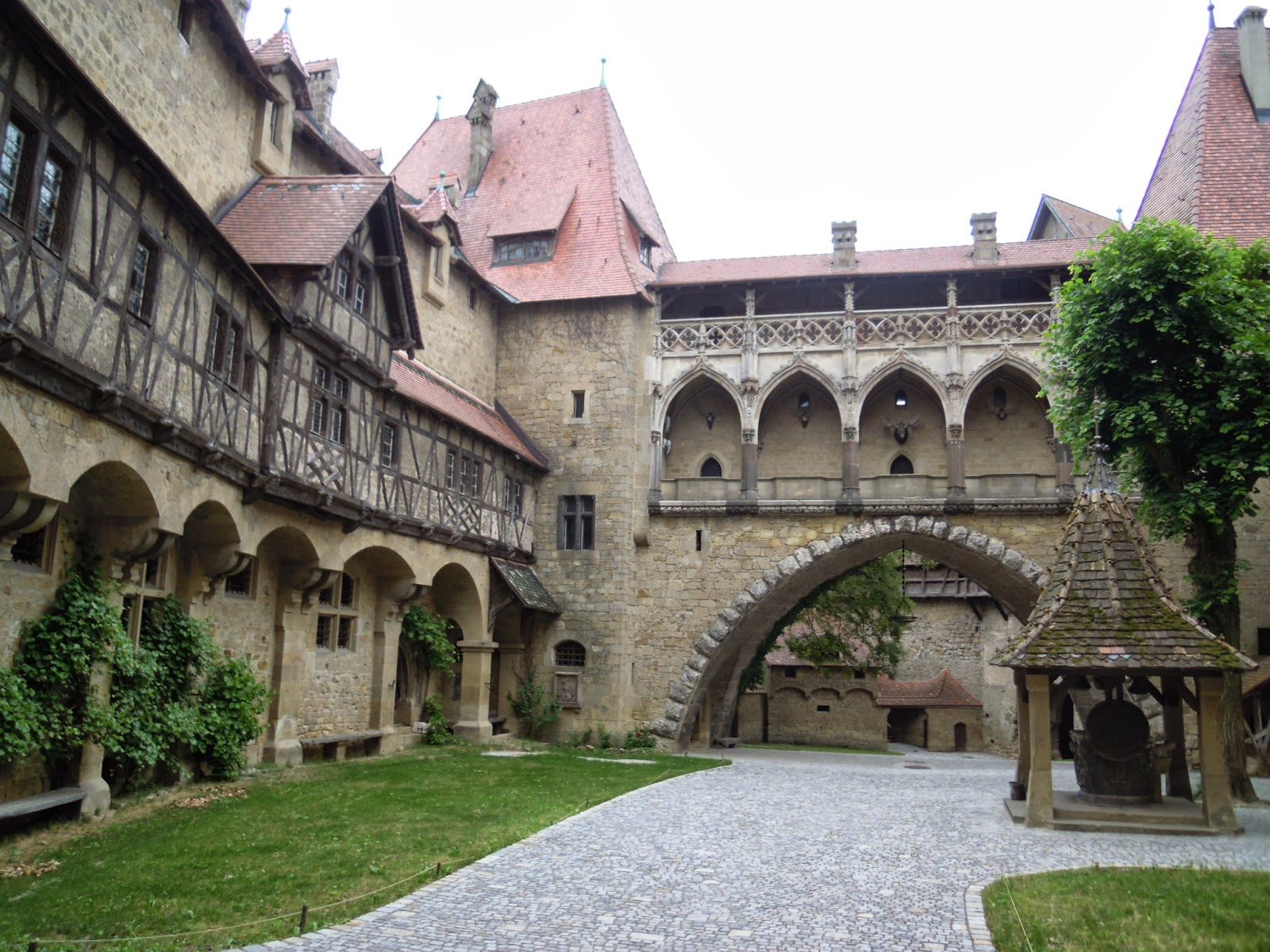This detailed photograph captures the courtyard of an old, rustic building that shares characteristics reminiscent of both English and French medieval architecture, predominantly evident in its Tudor style and cross-hatched mullioned windows. The building is constructed from sandy beige and dark brown sandstone, complemented by a red slate roof. The sky above is overcast, casting a cloudy and gloomy ambiance over the scene with no visible sunlight. The central focus of the image includes a cobblestone road flanked by bricks and patches of green grass on either side, leading to several low buildings connected by a series of archways. These buildings, at least three stories tall, feature elaborate stonework, including a small bridge with a balcony that links different parts of the structure. Notably, there is a small, pagoda-like shed with a tree behind it on the right, and a little red brick building housing a bell. The courtyard also contains a few bushes growing along the building's sides, emphasizing the antiquated and textured aesthetics of this historic manor or castle.